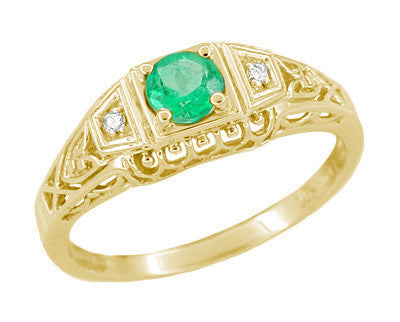This image is a close-up photograph of a magnificent woman's ring. The ring features a smooth gold band that widens at the top where it showcases a circular, light green, and transparent emerald held by four gold prongs. The centerpiece emerald has a very flat top, and on either side of this central stone, in separate squared-off settings, are two small diamonds. The upper third of the ring visible on the hand is adorned with intricate filigree, characterized by openwork gold allowing visibility of the underside. The entire front of the ring, including the sides of the band, is embellished with this delicate cut-out design, enhancing its elegant and exquisite appearance. The ring rests against a white background, emphasizing its gold, green, and diamond components.